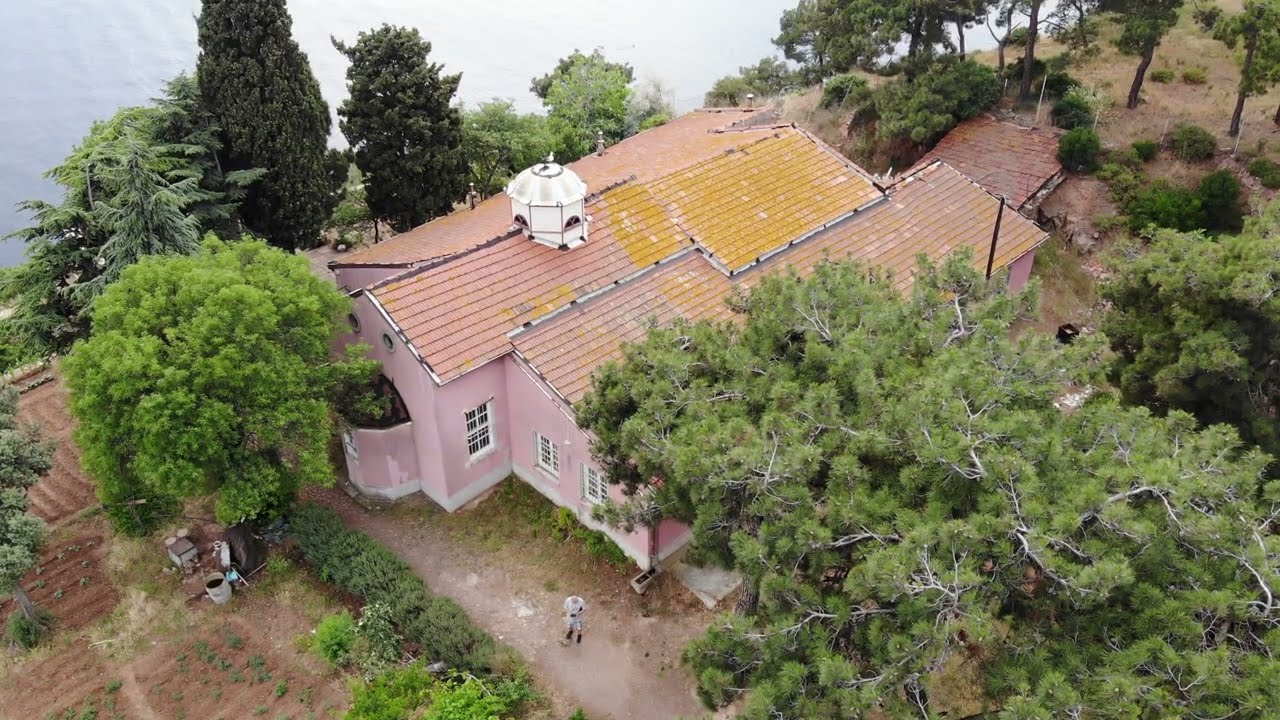This daytime aerial photograph captures a picturesque pink building, possibly a fancy house or a church, with a reddish-pink tile roof that shows about 40% coverage of yellow-green moss. The house, a one-story structure, features white stucco walls adorned with white-striped windows, and a noteworthy cylindrical, whitish structure with a dome on top, hinting at ecclesiastical architecture. Surrounded by a variety of trees in different shades of green, the house is divided into three sections: a main section with a triangular roof and two side sections with sloped roofs. In the foreground, a grassy area with patches of dirt is visible, where a man in a white shirt and shorts is seen potentially operating a drone. The scene includes a garden with soil stairs in the lower left corner and a wooden bridge or pier in the upper right. The location, likely perched on a hill, offers a view descending to a body of water, adding to the serene and beautiful lakeside or seaside atmosphere.